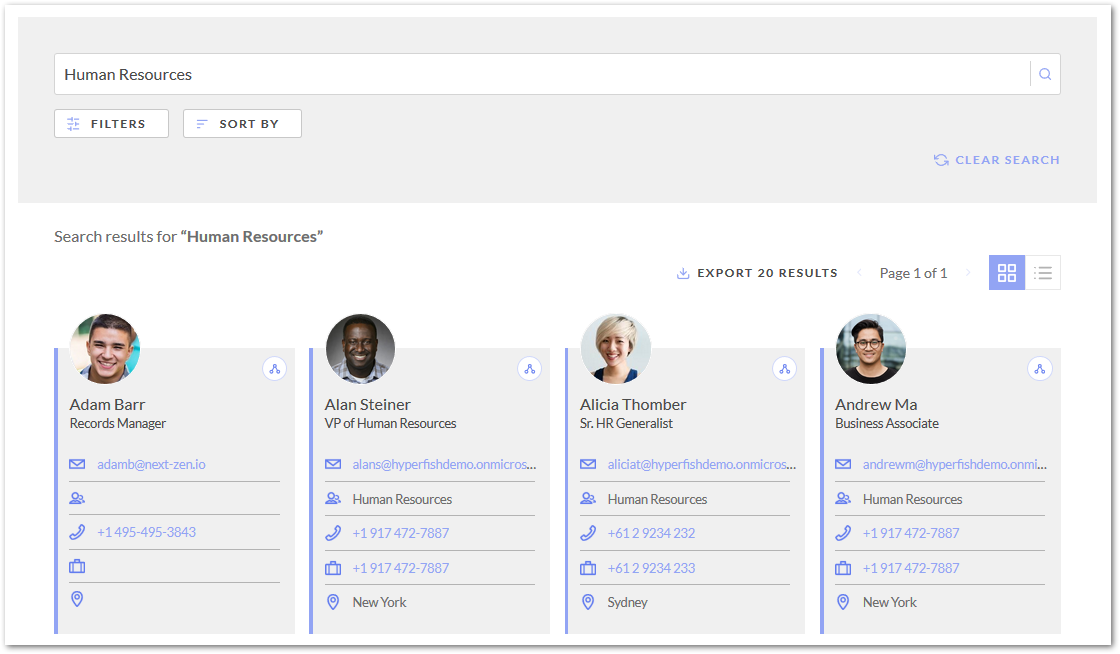The image depicts a user interface for a Human Resources search on a website. At the top of the screen, the search bar displays the term "human resources," flanked by filter options and a sorting function. To the right, a "Clear Search" button is situated within a gray rectangle. Below this section, the interface transitions to a white background, showcasing the search results for "human resources."

Users can export up to 20 results at a time and are currently viewing page one of one. The interface offers the option to display results either as tiles or in list format, with the current view set to tiles. Four individuals are featured in this layout: Adam Barr, Alan Steiner, Alicia Thomber, and Andrew Ma. Each person's profile is presented with a circular headshot, all smiling, followed by their name and role. These profiles are framed within a gray rectangle accentuated by a blue stripe down the side. Each entry includes an expandable section, accessible via a dropdown button, which reveals additional information.

From left to right, the details are as follows:
1. **Adam Barr**: Records Manager
2. **Alan Steiner**: Vice President of Human Resources
3. **Alicia Thomber**: Senior HR Generalist
4. **Andrew Ma**: Business Associate

Each profile also lists email addresses, phone numbers (sometimes multiple), and workplace locations. The meticulous design ensures all necessary contact information is readily accessible for each individual.